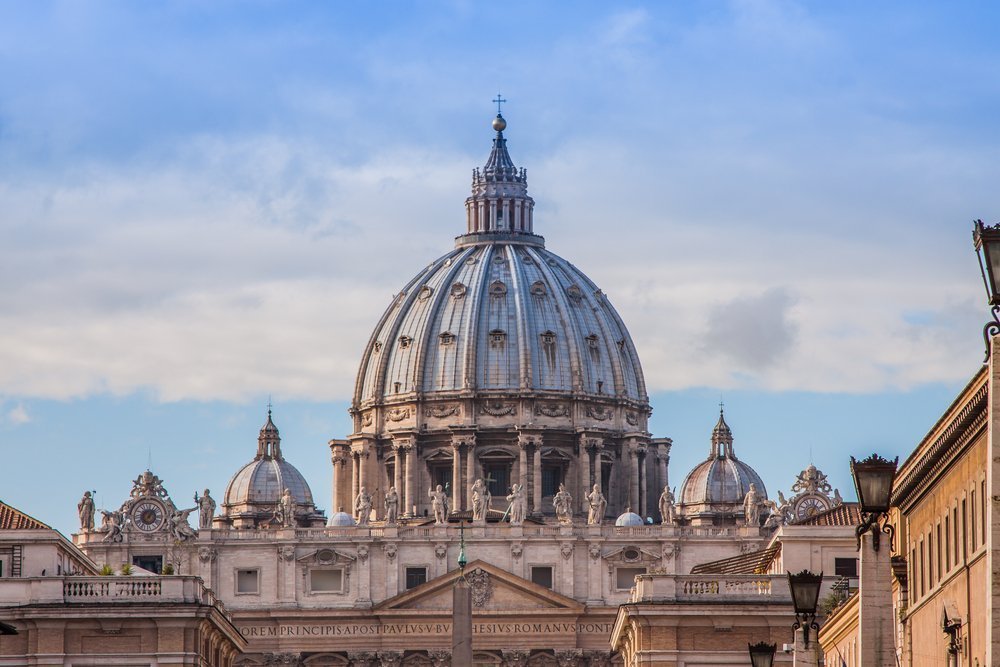The image showcases an impressive historical building characterized by its grand dome structure, topped with a cross. The dome, a focal point of the architecture, is flanked by smaller domes on either side, all adhering to Roman architectural principles with carved posts and pavils. Below the main dome, a line of statues is intricately carved into the building’s facade, depicting various figures or individuals, adding to its dignified appearance. A massive clock is prominently featured above a balcony, beneath the main entrance. At ground level, a row of buildings can be seen lined up on the right, illuminated by night lamps on either side, contributing to the serene and majestic ambiance. A hanging cloud starts at the base of the top dome, creating a light blue bar effect where the sky breaks through, adding to the striking view of this prestigious edifice.